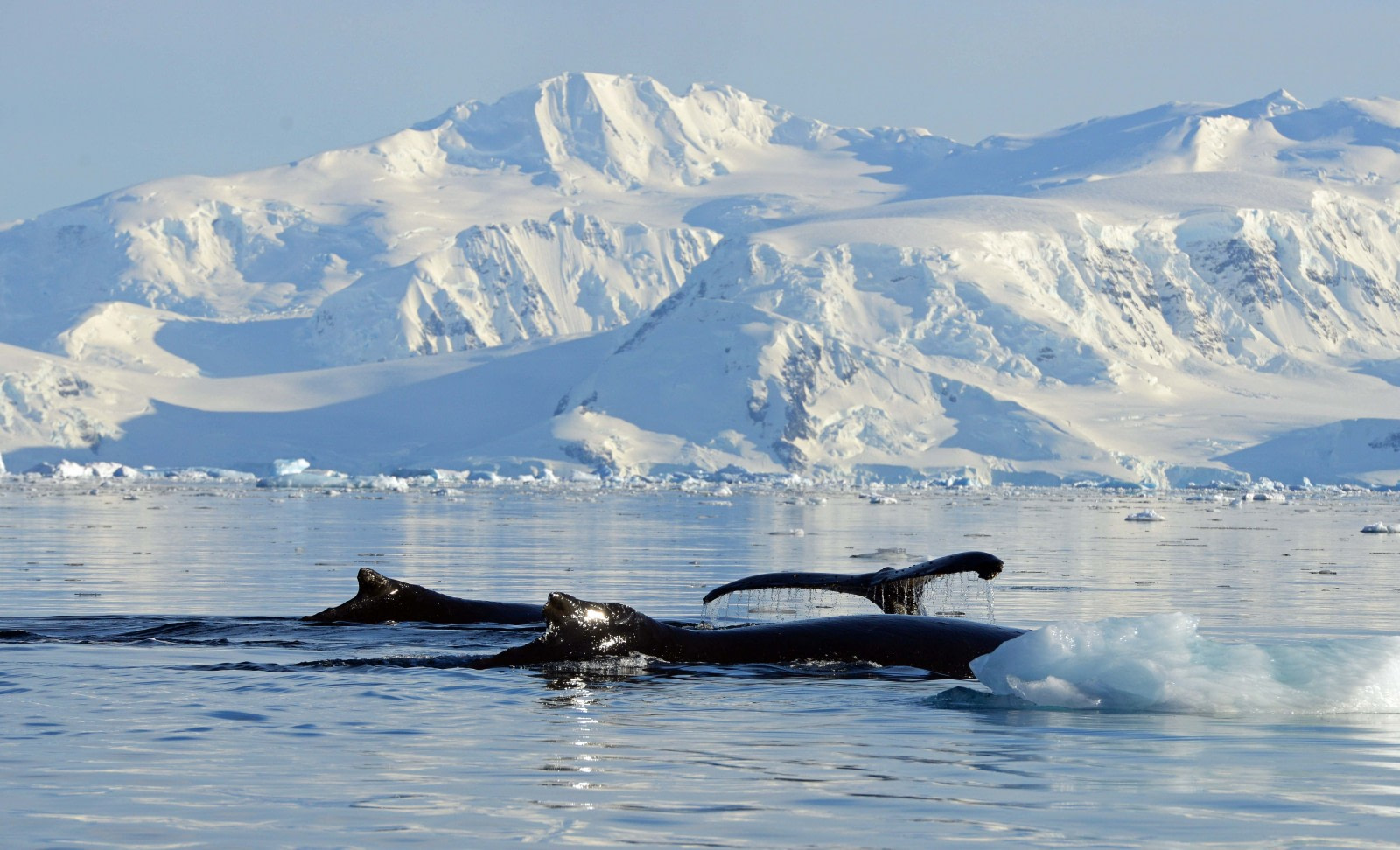In this vibrant and colorful photograph set in an arctic environment, a massive iceberg, mountainous in size, dominates the background, stretching from the upper left corner and extending towards the center before leveling off to the right. The iceberg is a stunning blend of white and blue hues at its peak, with a craggy surface descending towards the water. Smaller ice pieces, likely fallen from the glacier, float in the calm water below. The clear blue sky dotted with minimal clouds enhances the icy landscape, where everything appears blanketed in snow, rendering the rocks beneath invisible.

In the foreground of this serene bay scene, three black whales are visible near the water's surface. One whale’s tail and partial body are prominently displayed, while two others partially emerge with only their dorsal fins visible. Their presence contrasts strikingly with the icy, tranquil setting. Additionally, a wing-like structure or black platform, possibly part of a wrecked boat, is situated on a strip of land jutting from the water, adding an element of mystery to the scene. An isolated chunk of ice floats just above the right corner of the image, indicating the whale swimming past it. No other animals are present in this pristine and captivating arctic landscape.